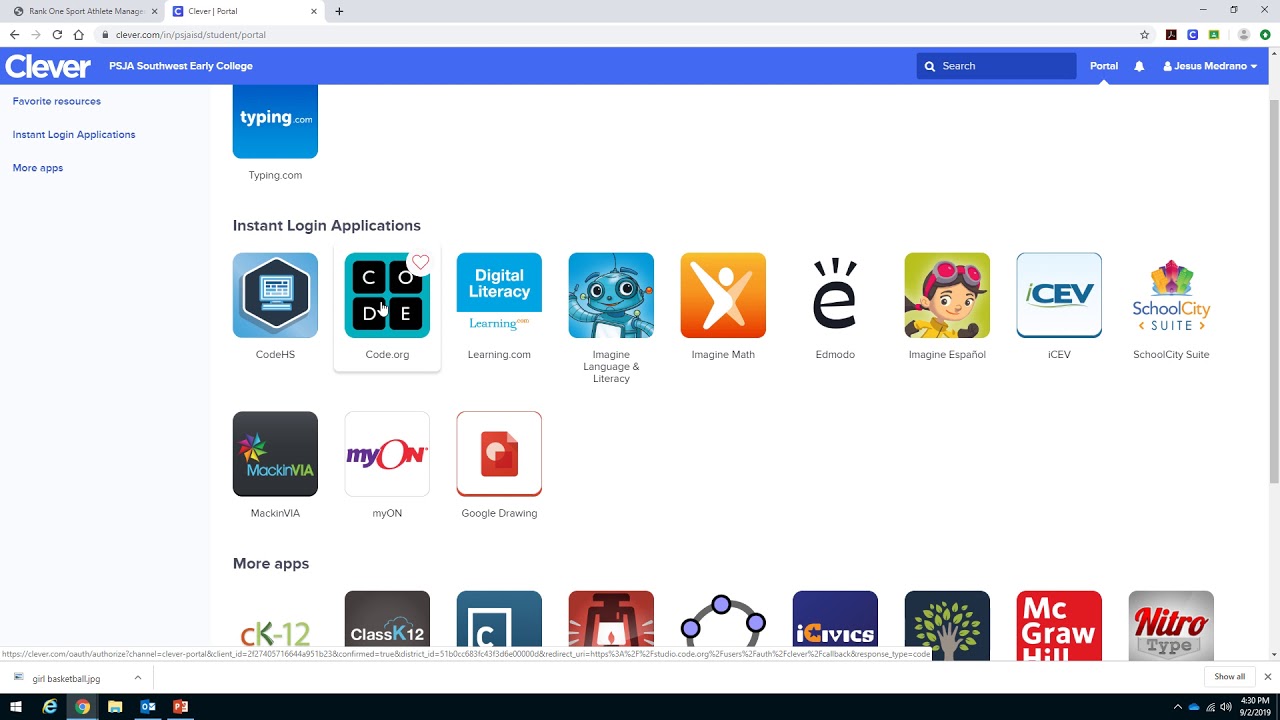The image captures a video of a Chrome browser window open to the Clever website, specifically tailored for PSJA Southwest Early College. The interface boasts a blue-themed design, emphasizing various sections such as "Favorite Resources," "Instant Login Applications," and "More Apps," all accessible via tabs located in the bottom left corner.

The main section of the webpage displays a diverse array of educational applications. These include Typing.com, CodeHS, Code.org, Learning.com, Imagine Language and Literacy, Imagine Math, Edmodo, Imagine Español, ICEV, SchoolCity Suite, Mac and VI, MyON, and Google Drawings. 

Towards the bottom, additional applications are listed, clearly geared towards enhancing academic performance and providing educational resources. These include CK-12, Class K-12, McGraw Hill, iCivics, and NitroType. 

The user logged into this educational portal is identified as Jesus Medrano. The surrounding desktop environment of the computer includes icons for Internet Explorer, Chrome, Files, Outlook, and PowerPoint, indicating a typical setup for educational or professional use. Additionally, a recently downloaded file named GetBasketball.jpg is visible among the browser's recent downloads.